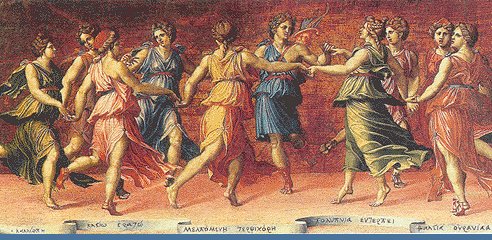The painting depicts a group of ten women, possibly with one man among them, engaging in a traditional dance on a stage. They form a circle, holding hands, their legs animated as they move in rhythm. Each dancer is adorned in vibrant robes of orange, green, blue, yellow, white, and other colors, reminiscent of Grecian attire, with various colored headdresses. The setting features a red background and an orange-brown floor, which suggests they are performing on a stage. At the bottom edge of the image, there are white banners with Greek lettering, possibly labeling each dancer. The scene is bathed in stage lights, adding a sense of drama and focus to their dynamic movement. This horizontal rectangular painting, evocative of a Renaissance fresco, captures the lively essence of the dancers in vivid detail.